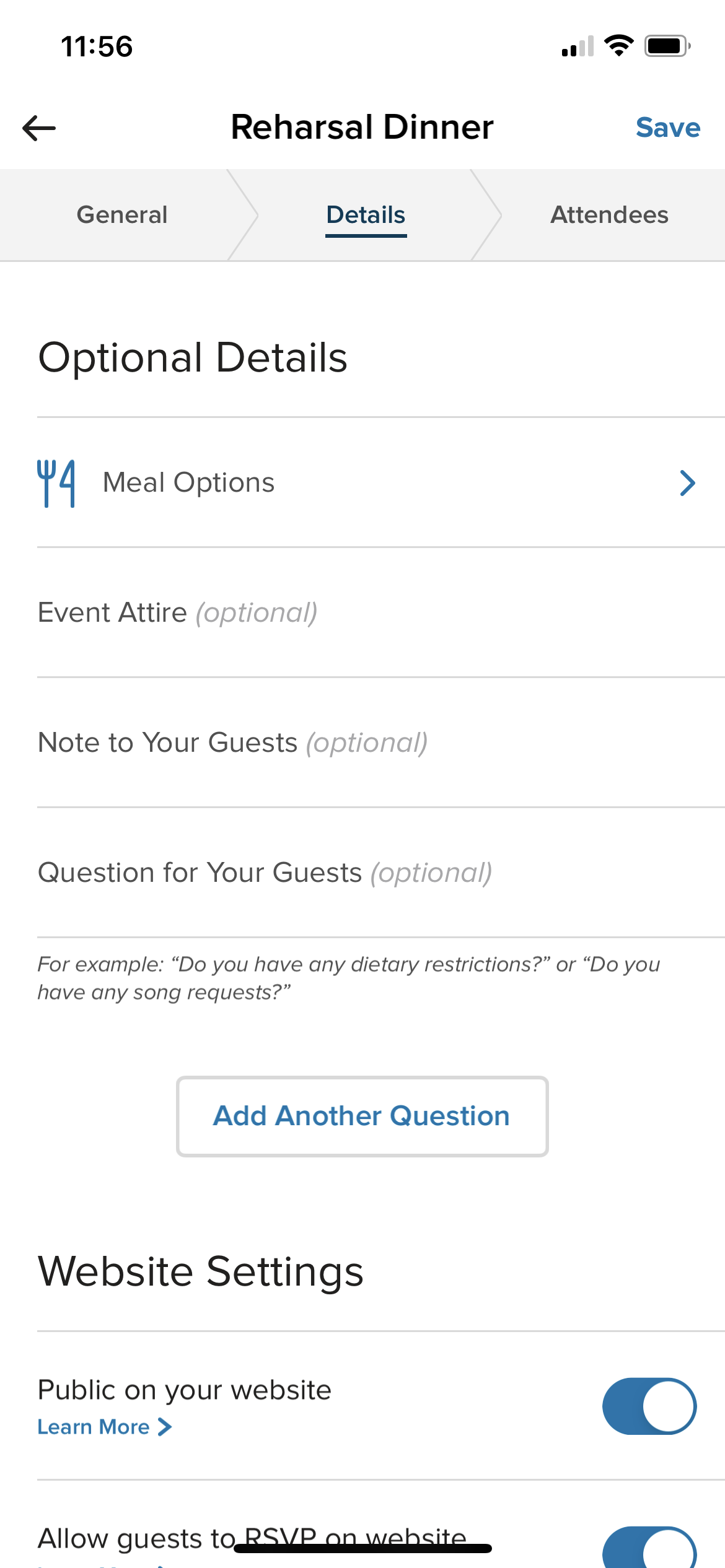A screenshot displays a wedding planning app, specifically showcasing a section dedicated to the rehearsal dinner. The top of the screen prominently features the title "Rehearsal Dinner," indicating that this section provides detailed plans and information about the event. The app is designed to facilitate communication and planning for weddings, allowing users to send important details via text message or within the app.

The interface includes fields for "General Details" and "Attendees," along with "Optional Details" such as meal options, event attire, notes to guests, and questions for guests. Users have the ability to add custom questions, for example, asking guests about dietary restrictions or song requests for the event. 

The app also includes settings to make the information public on a website and allows guests to RSVP directly through the site. The predominantly white interface is accentuated with blue icons, providing a clean and user-friendly design. Overall, the app offers comprehensive tools for planning a wedding or similarly significant event, ensuring that all details are easily accessible and modifiable.